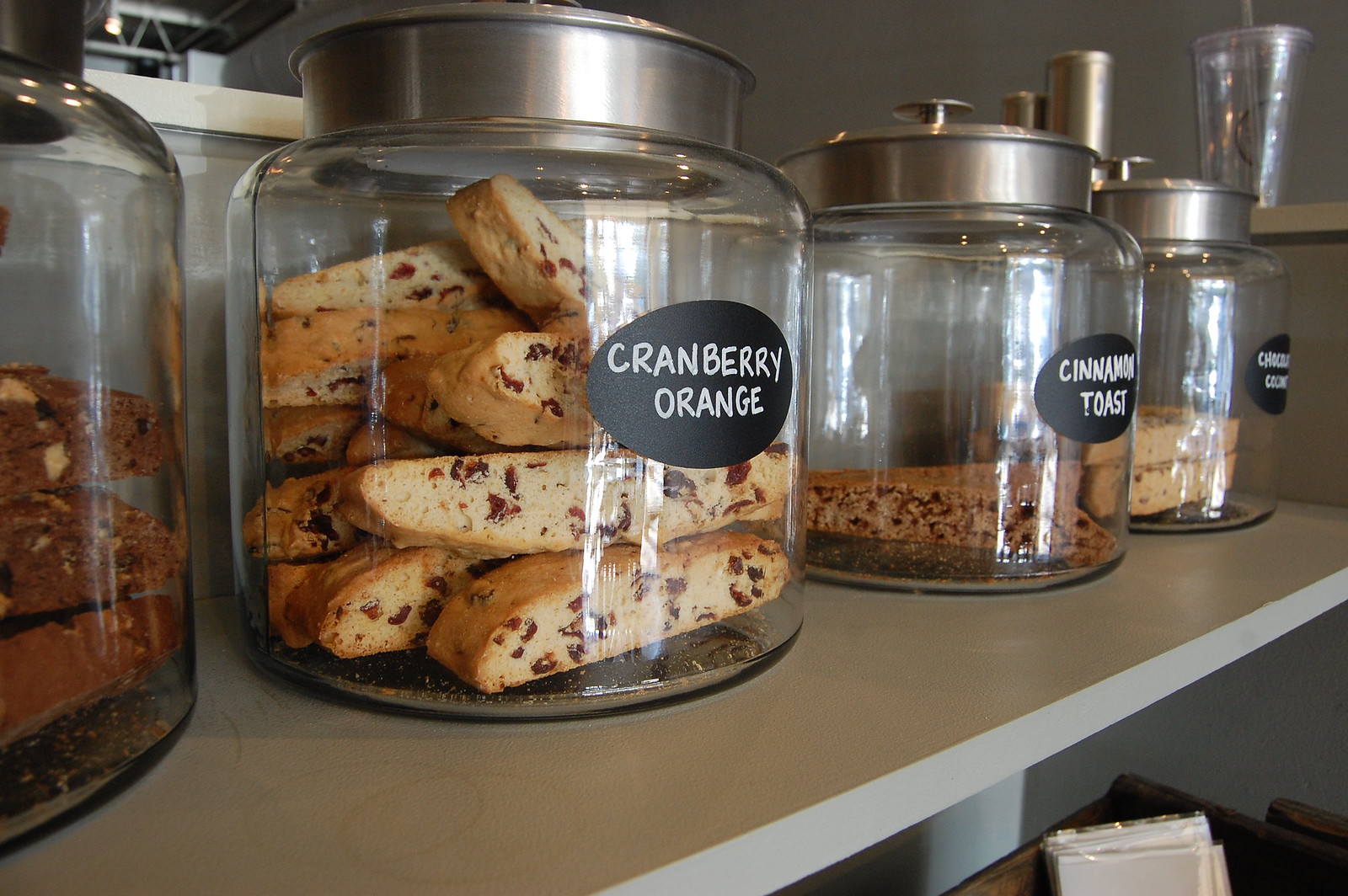The image shows four large, clear glass jars with round-handled silver lids arranged on a light gray shelf. The first jar on the left is partially cut off, revealing what appears to be chocolate-flavored scones. The next jar features a black label with white chalky letters reading "cranberry orange," and is filled nearly to the top with lighter-colored scones. The third jar, labeled "cinnamon toast," contains a single darker scone. The fourth jar, holding two lighter scones, has a label that reads "chocolate chip cookie." Below this shelf, there is a partially visible darker gray bin with white items stacked inside.